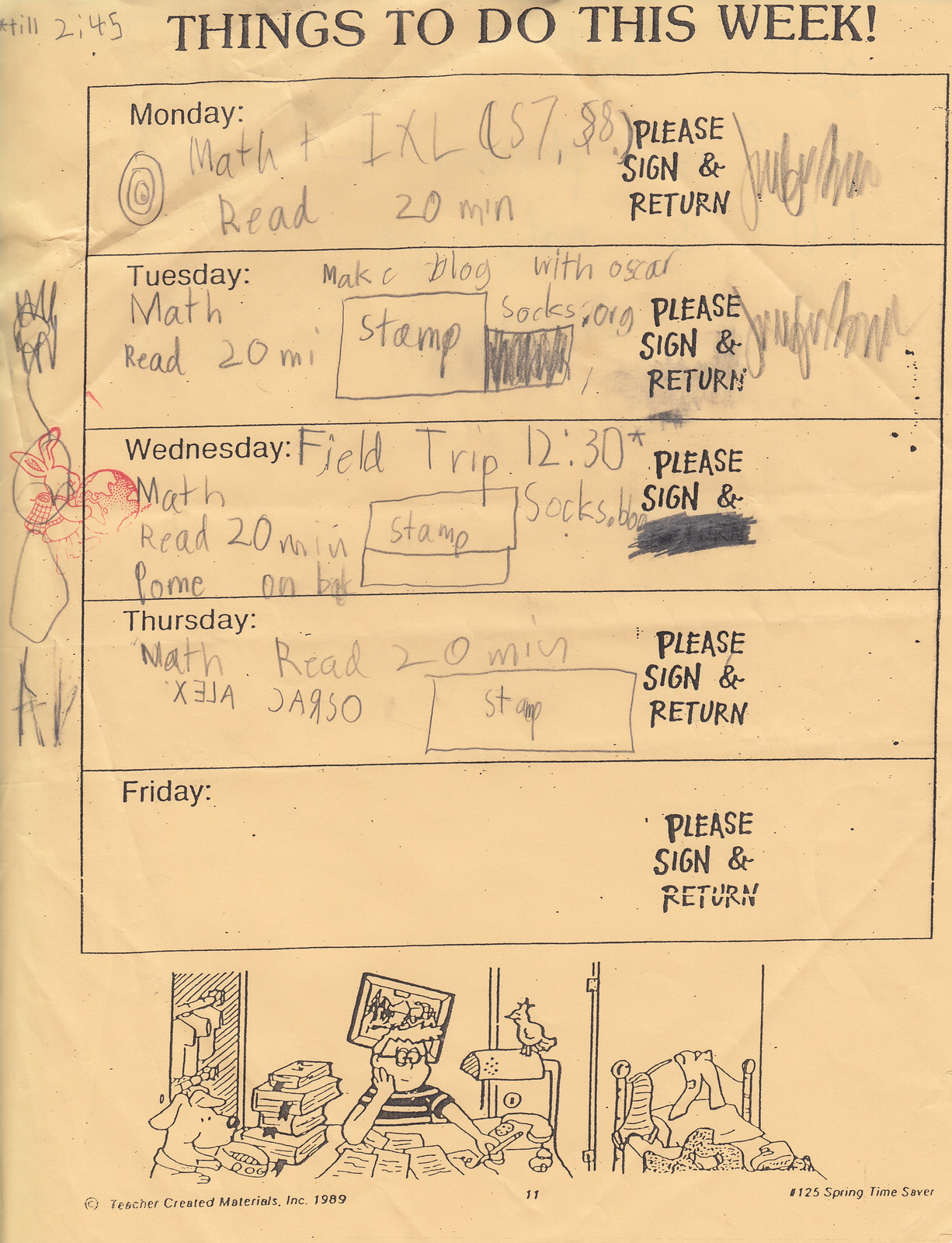The image shows a student's weekly schedule on a green-yellow notepad titled "Things to do this week!" The page is divided into five vertical rectangles, each dedicated to a day of the week from Monday to Friday. 

- **Monday**: In a child's handwriting, the tasks listed are "Math, read 20 minutes, IXL (possibly s 7.88 or $7.88)." There is also a note "Please sign and return," accompanied by a scribbled signature.
- **Tuesday**: Lists "Math, read 20 minutes," and includes a handwritten box with "Stamp." There's also a note about "Make blog with socks org," and again, "Please sign and return," with a scribble signature.
- **Wednesday**: The tasks are "Field trip 12:30," "socks.org," "Stamp" in a box, "Math, read 20 minutes," although the text is difficult to read.
- **Thursday**: Repeats "Math, read 20 minutes," and "Stamp" in a box.
- **Friday**: No tasks are listed.

On the left margin, there is a doodle resembling a stylized cat. At the bottom of the page, there is a cartoon illustration depicting a child in a striped polo shirt, sitting at a desk doing homework, with various school-related items around him. The setting includes open books, a crooked painting, a lamp with a bird on it, and scattered clothes, suggesting a typical, slightly messy student's room.